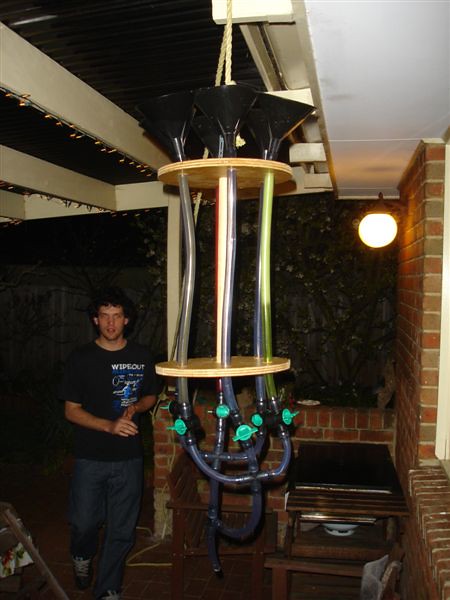This is a detailed nighttime color photograph taken outdoors, presumably on the patio or porch of someone's backyard. The scene is centered around a unique homemade contraption suspended from the white ceiling molding. This intriguing device features black funnels at the top, connected to rubber hoses that descend into tan wooden circles, with green nozzles at various points, suggesting it controls some kind of liquid or gas flow.

To the left of the contraption stands a person, likely a man, dressed in a black t-shirt with the words "Wipe Out" in white letters, blue jeans, and sneakers. He has medium-length dark curly hair and is standing with his hands positioned in front of him, his right hand touching the fingers of his left. His posture suggests a relaxed interest in the device next to him.

The setting reveals additional details: a backdrop of green trees indicating a suburban backyard, and a red-bricked patio ground. Other items include a wooden table and a chair, enhancing the cozy ambiance of the scene. The brick walls suggest the exterior of the house, and a porch light illuminates the setting modestly, adding to the nighttime atmosphere. A circular light bulb, possibly a sconce, can be seen on the right edge of the photo, and there seem to be small lights strung up nearby, contributing to the overall warm and inviting atmosphere.